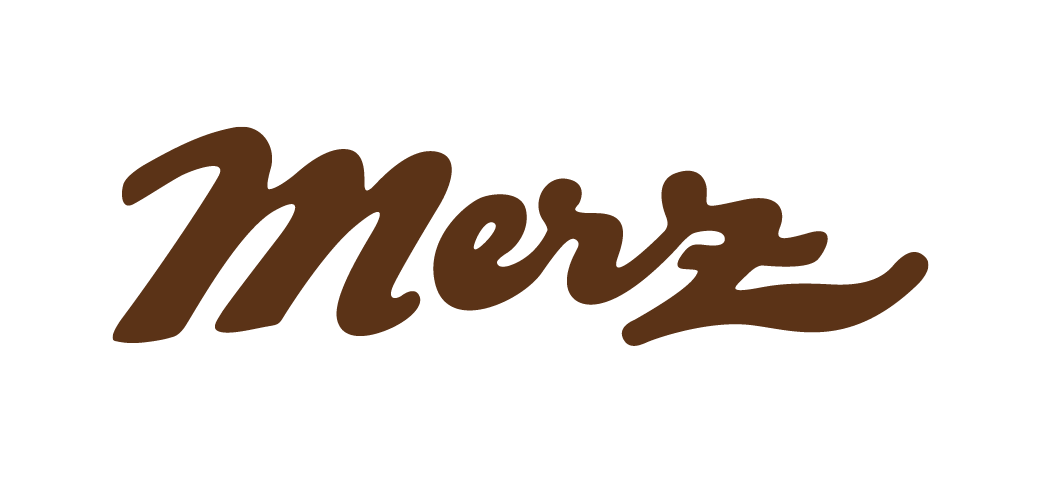The image features the text "MERZ" rendered in cursive with dark maroon, almost brown, thick lettering. The capital "M" is distinct and not connected to the "E," while the "E," "R," and "Z" are linked in an elegant, fancier cursive font. The text is fairly large, approximately an inch and a half tall by six inches wide, and centered on a stark white background. There are no additional elements or images in the picture, making the simple yet bold text the focus. The capital "M" is roughly half the size of a pointer finger, providing a sense of scale.